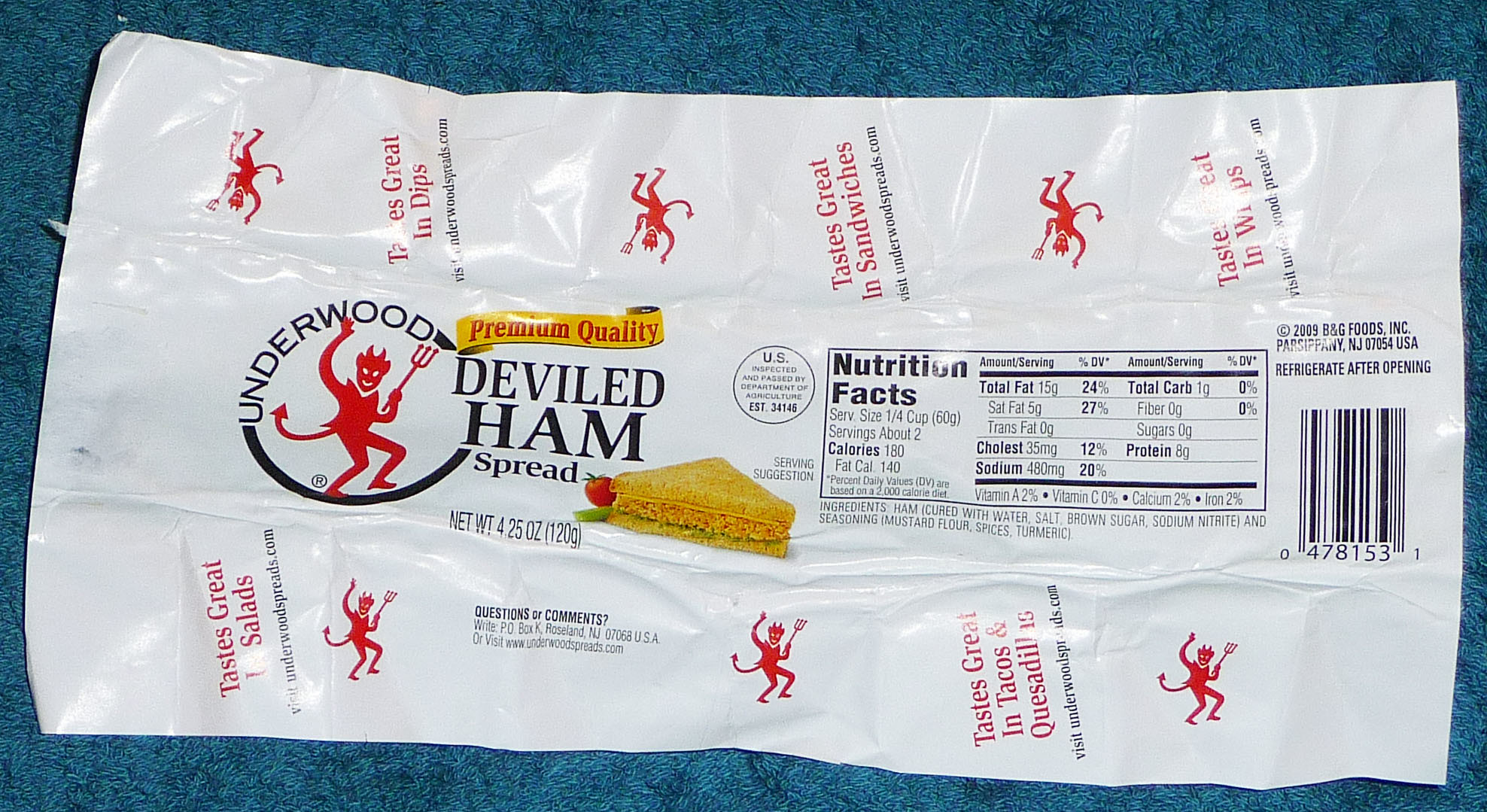This photograph captures a flattened wrapper of Underwood Deviled Ham Spread, originally designed to encase a can of the product. Laid out against a blue, textured background resembling a sweatshirt, the white wrapper prominently features the Underwood branding. 

On the left-hand side, the name "Underwood" is printed in black letters within a circular emblem. This circle is half black and showcases the iconic Underwood devil clutching his pitchfork, complete with a forked tail. Adjacent to the emblem, a yellow sign with red lettering declares "Premium Quality," followed by the product name in various styles: "DEVILED HAM" in all capital letters, "HAM" in bold font, and "spread" below in standard text. The weight of the product is also indicated as "Net Wt 4.25 oz (120 g)."

To complement the textual elements, a small illustration of a sandwich filled with deviled ham is depicted, accompanied by a tomato slice to its left. 

On the right side of the wrapper, the nutrition facts panel lists essential data: a serving size of a quarter cup, approximately two servings per container, 180 calories per serving with 140 calories from fat. Below this, a barcode is situated with instructions above it to "Refrigerate After Opening," and the manufacturer's details: "2009 B&G Foods, Inc., Parsippany, NJ 07054 USA."

Encircling the outer edges of the wrapper, the phrase "Tastes great in" is repeated six times, each followed by a different suggestion: salads, dips, sandwiches, tacos and quesadillas, and wraps. Below each recommendation, respective websites "visitunderwood.com" or "visitunderwoodspreads.com" are listed, along with a repeating motif of the little devil in red. 

The intricate design not only reinforces the brand identity but also provides versatile serving ideas, ensuring the wrapper is both functional and engaging.